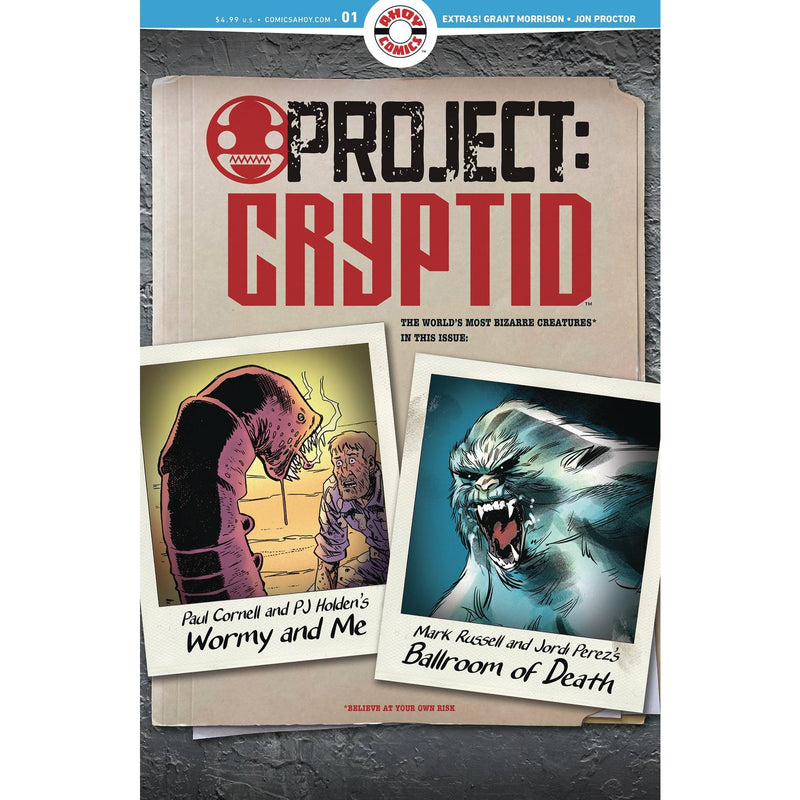This detailed comic book cover features a thematic design that emulates a detective dossier. At the very top, a light blue strip displays white text listing the price as $4.99 U.S. and includes the website “comicsahoy.com,” along with “Number 1” and “Extras: Grant Morrison, John Proctor.” Centered below this strip is a white circle with "Ahoy Comics" printed in bold red. The main background of the cover is a stony gray texture, overlaid by a large manila folder prominently titled "Project Cryptid" in striking black and red text. Below this, it reads, "The world's most bizarre creatures in this issue."

The manila folder appears to hold two Polaroid photographs. The left Polaroid depicts an alien-like worm with sharp teeth, appearing ready to attack a man. Underneath, it is labeled "Paul Cornell and PJ Holden's Wormy Enemy" in black text. The right Polaroid shows a menacing, white fur-covered Yeti-like creature with huge fangs and black eyes with tiny white pupils, labeled "Mark Russell and Jordi Perez's Ballroom of Death" in black text below.

At the bottom of the manila folder, in small, fine red print, it reads, "Believe at Your Own Risk." The overall design mimics an eclectic investigative report on mythical creatures, rendered in a comic book style.